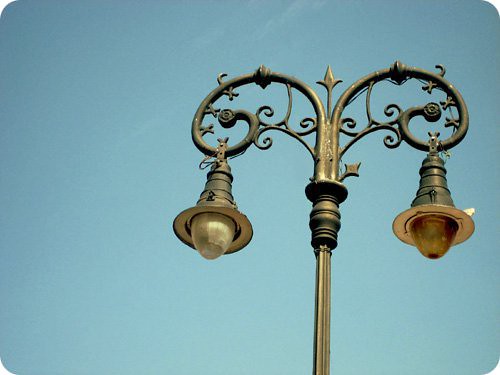The image depicts a slightly wider-than-tall photo with rounded edges, featuring a vintage street lamp set against a light teal sky. The sky is mostly solid in color, perhaps a bit darker at the edges, creating a serene backdrop for the ornate street light. The street lamp, appearing well-worn with some rust, showcases an intricate, artistic design. The thin, black wrought iron pole rises and splits into two decorative loops resembling ram horns or vines. Each loop supports a lantern-like light, shaped like inverted bells or glass domes, hanging delicately. Given the daylight setting, the actual brightness of the bulbs isn't visible, but the overall scene captures a moment of timeless beauty under a clear, sunlit sky.